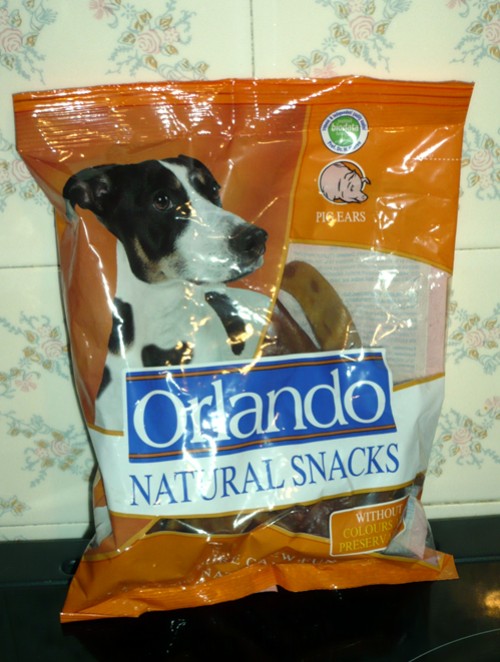The landscape-oriented, color photograph captures an orange and clear package of dog snacks, particularly pig ears, which is positioned at a 90-degree angle to the right. To read the text properly, one must tilt their head to the right. The bag features the brand name "Orlando" prominently in white text within a blue rectangle, set inside a large white rectangle. Above and to the left of the brand name is an image of a black and white dog with a white snout and brown spots, gazing upward. Below "Orlando," it reads "Natural Snacks" in blue font, and further specifies the contents as pig ears with a small cartoon of a pig in the top right corner within a white-bordered circle. The packaging, which appears unopened, reveals chewy, brown snacks inside. The background consists of white tiles adorned with pink and green floral patterns, likely on a kitchen counter, indicated by the grey grout lines between the tiles. The image is well-lit, with noticeable reflections—possibly from a camera flash or another light source—on the package.